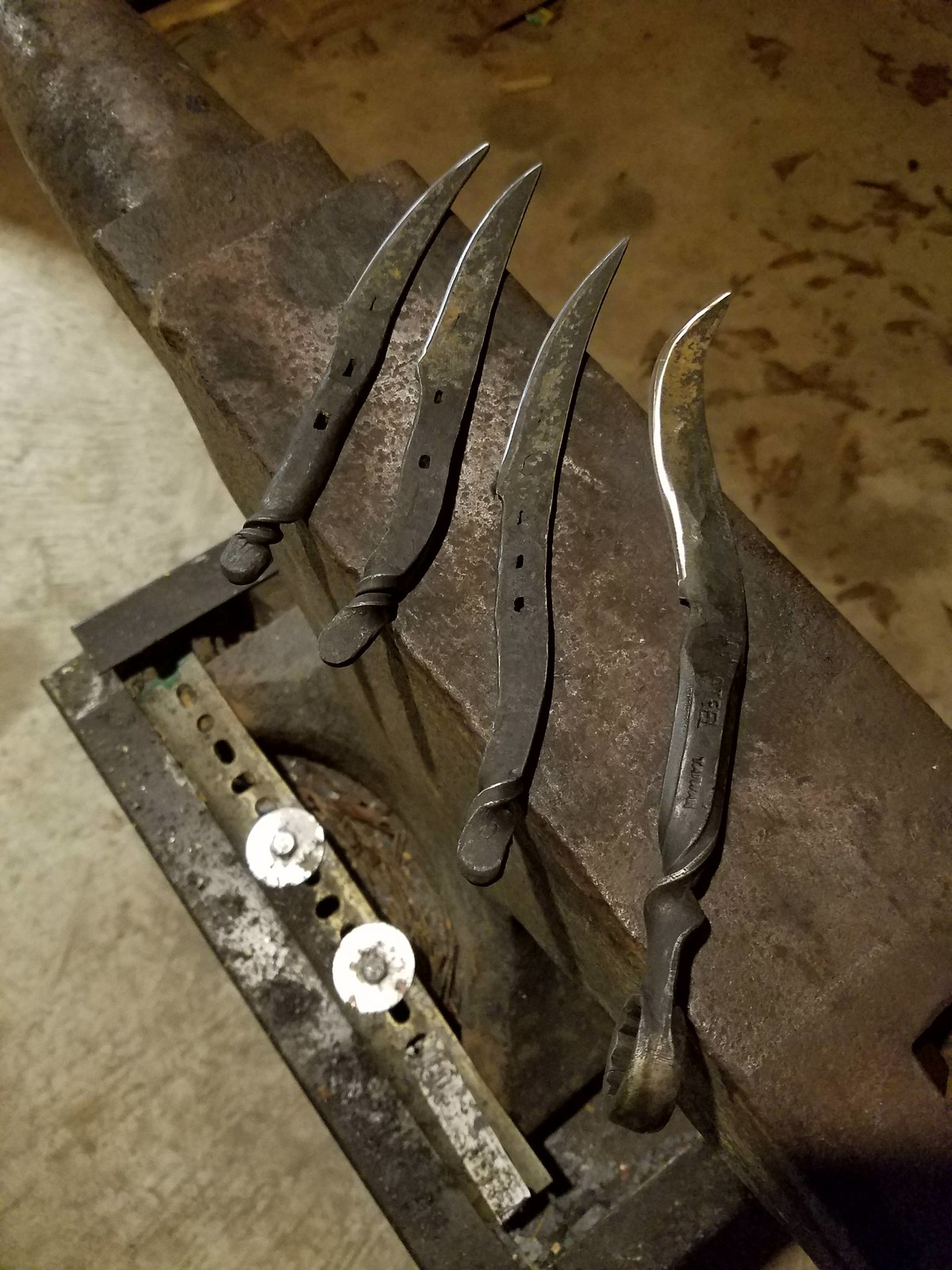The image depicts a light brown, tan workbench that serves as the focal point, topped with an array of tools and blades. Prominently positioned on the worn edge of the workbench are two ancient, rusted cleavers, their silver surfaces only faintly visible through the corrosion, likely aging over 50 years. Resting atop these cleavers are four distinct blades of varying lengths. The smallest blade is on the left, followed sequentially by blades of increasing size, with the rightmost being the longest. Each blade features intricate craftsmanship, with some exhibiting a twist pattern at the end, possibly indicating they were crafted from repurposed wrenches, particularly the longest blade which retains the characteristic star-shaped opening of a wrench.

Additionally, off the table, there’s a glimpse of adjoining metallic machinery, though its precise function remains indeterminate due to the angle. To the side, an anvil sits heavily, utilized by blacksmiths, and part of the machinery includes a bar with large washers and bolts securing it. The workspace floor is a pale concrete, enhancing the industrial, workshop atmosphere of the scene. These blades appear recently sharpened and potentially await handle attachment, capturing a snapshot of ongoing craftsmanship and metalworking.